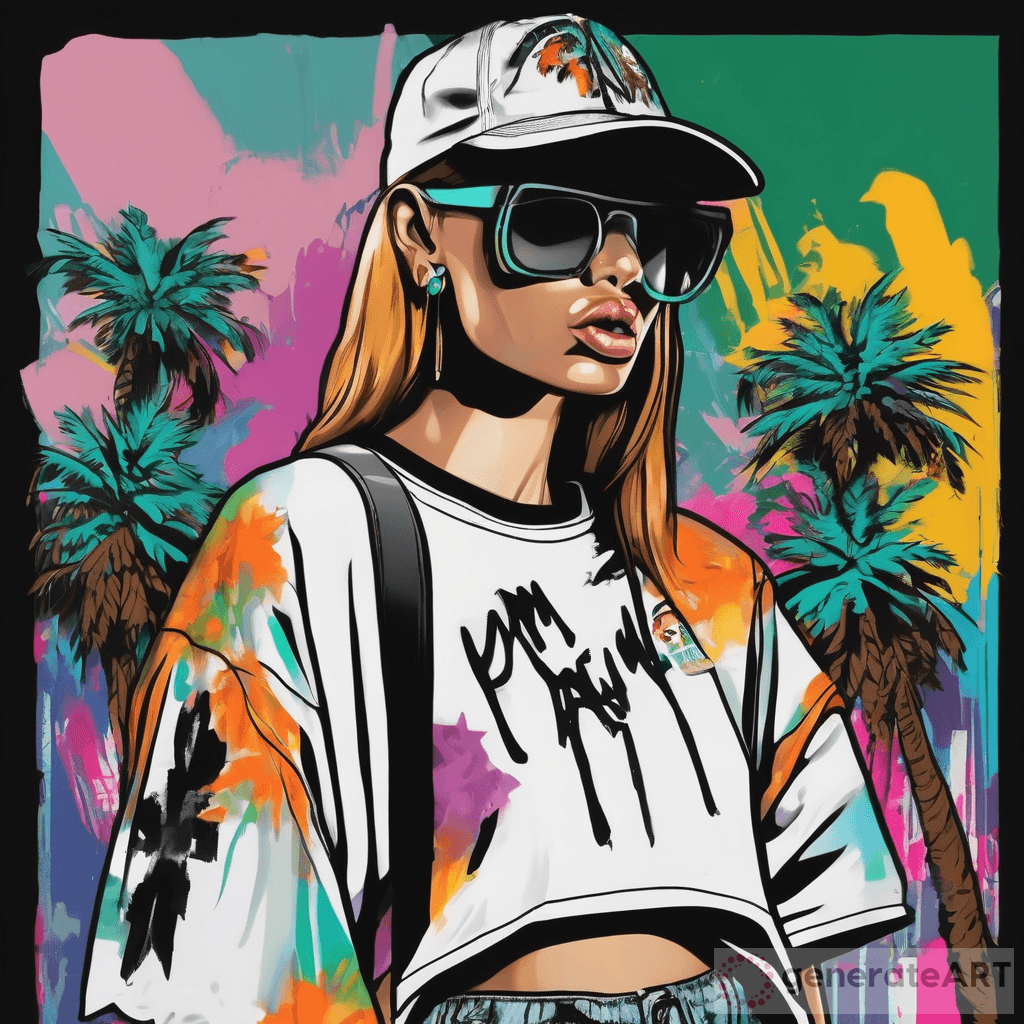This vibrant piece of pop art, reminiscent of 90s or early 2000s aesthetics, features a young girl as its focal point. She sports a tan complexion and orangish-blonde hair, adorned with a white hat decorated with a colorful design that matches her crop top. The crop top itself is white, splashed with hues of orange, black, yellow, blue, and purple, resembling a tie-dye or abstract pattern. She accessorizes with teal sunglasses and matching teal earrings, adding to her striking appearance. While the image cuts off at her waist, she appears to be wearing jeans.

The background is a visually stimulating mix of colors, with an artistic blend of green, blue, and splotches of pink and yellow. On the right side, a set of palm trees stands with a yellow splash, while two more palm trees with shades of pink and darker pink stand on the left. The overall scene exudes an energetic, retro vibe akin to something from Grand Theft Auto, marked by its bold palette and dynamic arrangement.